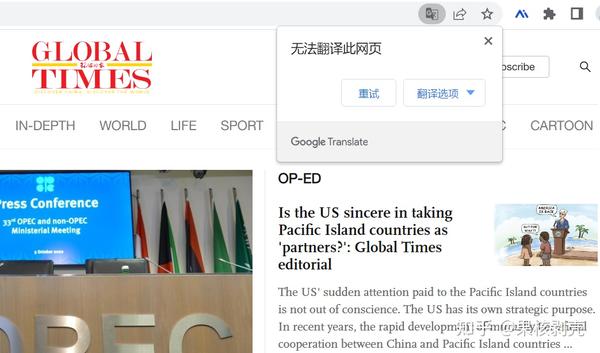On the screen, an article from the "Global Times" news website is displayed, categorized under news, in-depth, world, life, and sport. The featured image shows a press conference from the 33rd OPEC and non-OPEC Ministerial Meeting, with several flags visible in the background. The prominent headline reads "Is the U.S. sincere in taking Pacific Island countries as partners?" An editorial from Global Times suggests that the U.S.’ sudden interest in the Pacific Island countries is driven by strategic purposes rather than genuine concern, especially in light of the rapid military and technological cooperation between China and these nations.